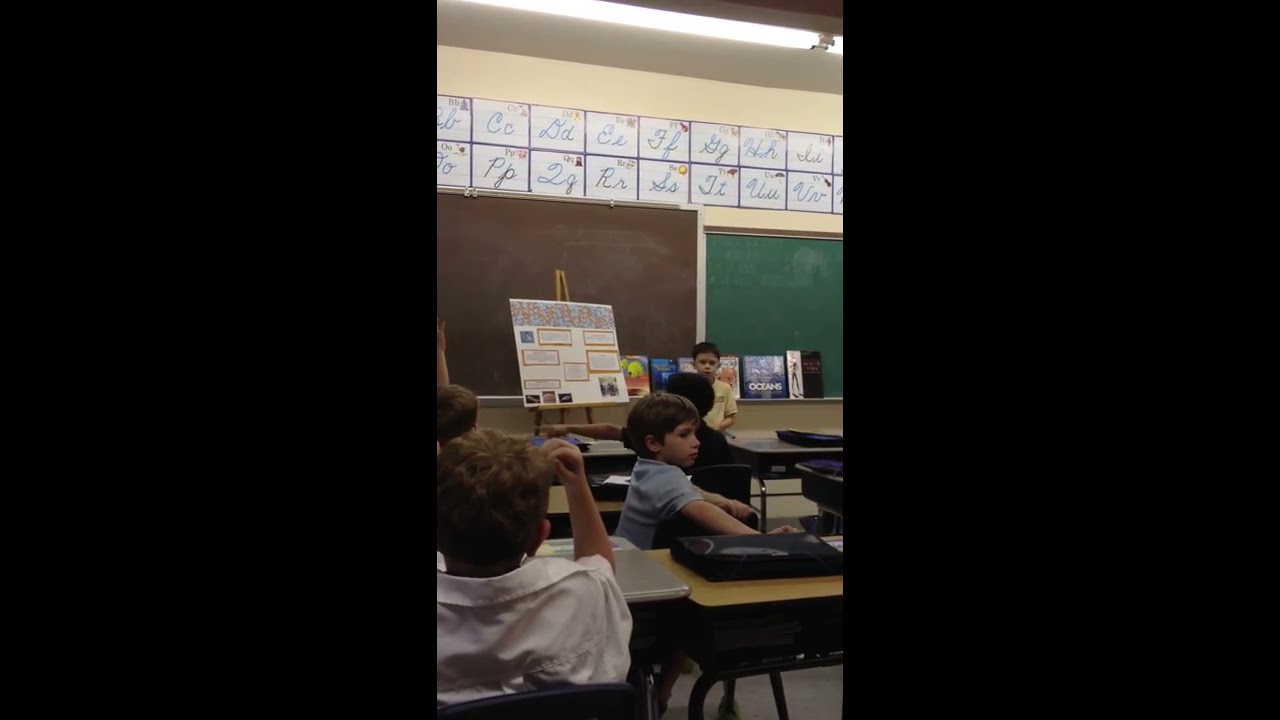This photo was taken inside a classroom and is split into three equal parts, with solid black segments on each side. The central part of the photo shows the back of a classroom, facing the front. There are five children in the image: four of them are sitting at their desks, with one child turned slightly to the right, wearing a blue t-shirt, and having medium-length brown hair. Another child, standing at the front of the classroom, is wearing a yellow t-shirt and has short black hair. It appears that he might be giving a presentation, as he stands next to a poster board, possibly explaining a project. Behind him, a black chalkboard is positioned on the left and a green chalkboard is on the right, both lined with about six children's books on their rails. The wall above the chalkboards features two rows displaying the alphabet in both uppercase and lowercase cursive letters. The atmosphere suggests a typical classroom setting, complete with binders and trapper keepers on the desks.